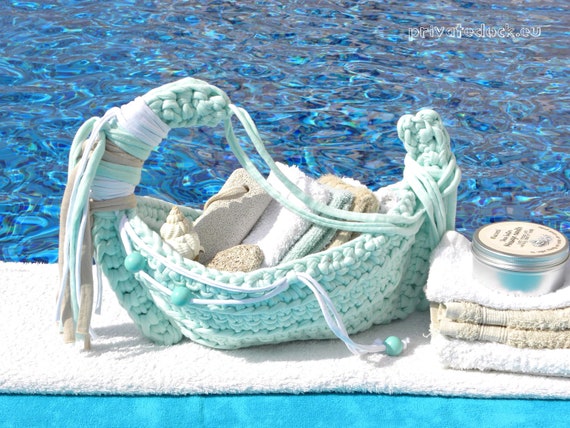The photograph captures a meticulously knitted basket shaped like a curved boat, composed of turquoise green yarn. The basket features a prow at one end and has brown, green, and white straps hanging from it. Nestled inside the basket are multiple terry cloth towels in shades of brown, white, and green, and a decorative conch-shaped seashell. The basket rests atop a white towel, situated on what appears to be a ledge. To the right of the basket, there is an orderly stack of additional towels—white and tan—capped with a small, metallic silver tin. In the background, the scene is completed by the clear blue expanse of a swimming pool, and the image is marked with the white text "Private Doc EU" in the top right corner.